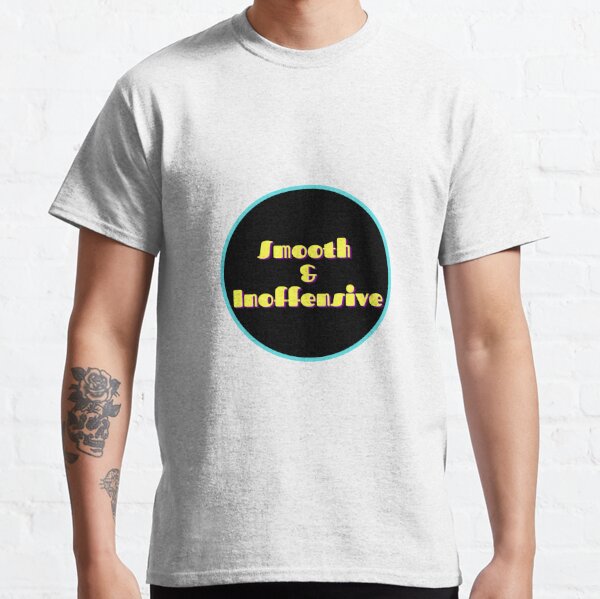The image showcases a detailed close-up photograph of a Caucasian man from the neck down to below the waistline, with the top of his head cropped out. He is wearing a light gray t-shirt that features a prominent design at the center. The design consists of a black circle outlined in a teal turquoise color. Inside the circle, the words "smooth & inoffensive" are displayed in yellow, retro-style font reminiscent of the 70s or 80s. The man has tattoos on his left arm, most notably a skull adorned with flowers and leaves on the lower part of his forearm. The clarity of the image is outstanding, with bright and even lighting highlighting both the t-shirt design and the tattoo details against the man's lighter skin complexion. The man's arms are relaxed by his waist, further emphasizing the t-shirt’s design and his tattoos.